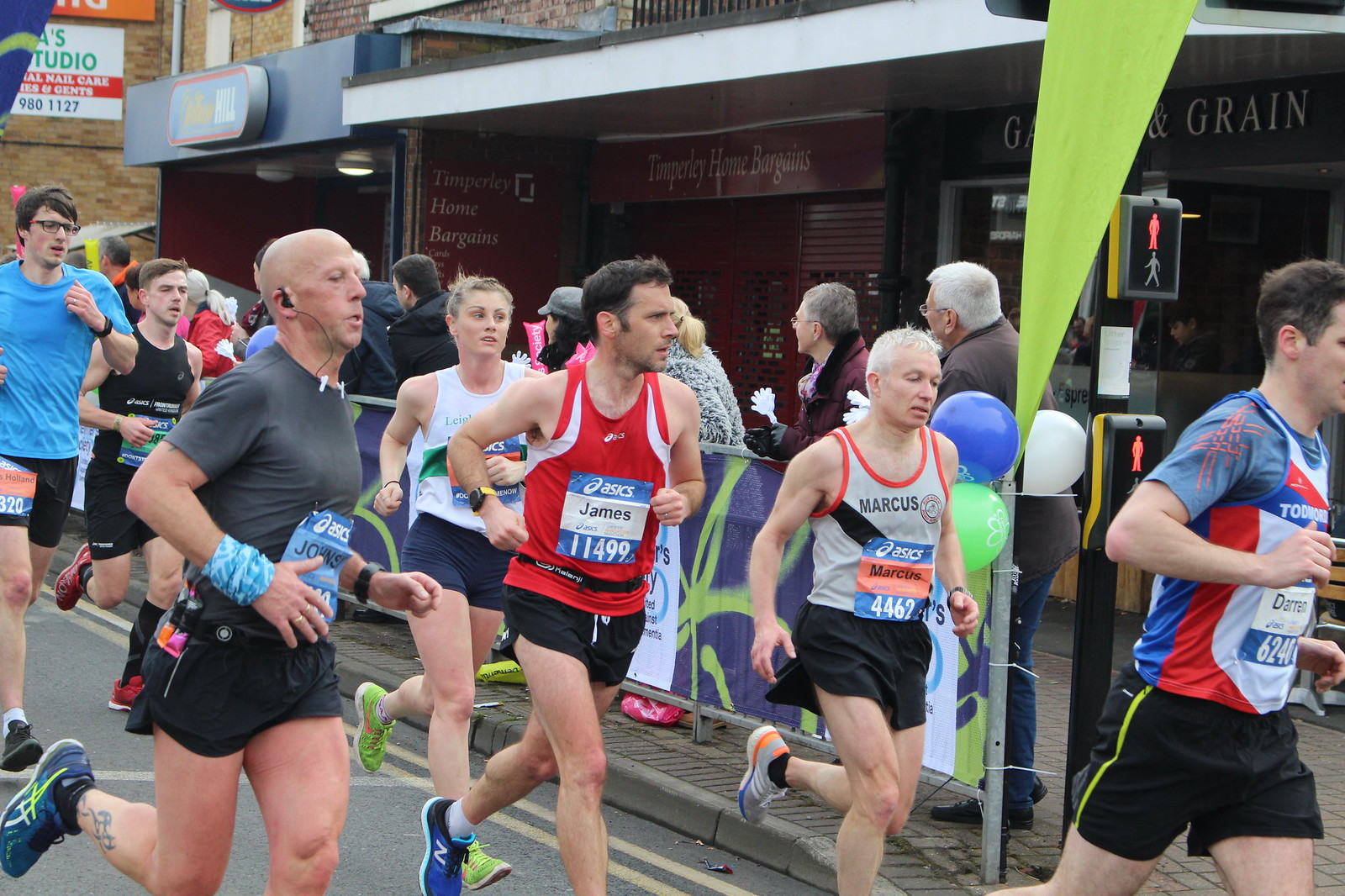The image depicts a marathon in progress featuring seven runners, predominantly men with one woman, all donning athletic clothing and sporting blue and white race numbers sponsored by ASICS. The runners, including one identified as James with bib number 11499, are captured mid-stride, heading towards the right side of the frame. In the bustling city backdrop, enthusiastic spectators line the sidewalk behind a barrier, cheering on the participants. The area is adorned with blue, green, and white balloons, signifying a festive atmosphere. Additionally, storefronts with visible signage are present, and a pedestrian walk/stop signal is noticed to the right. The collective enthusiasm of the crowd and the vibrant decorations highlight the event's celebratory nature.